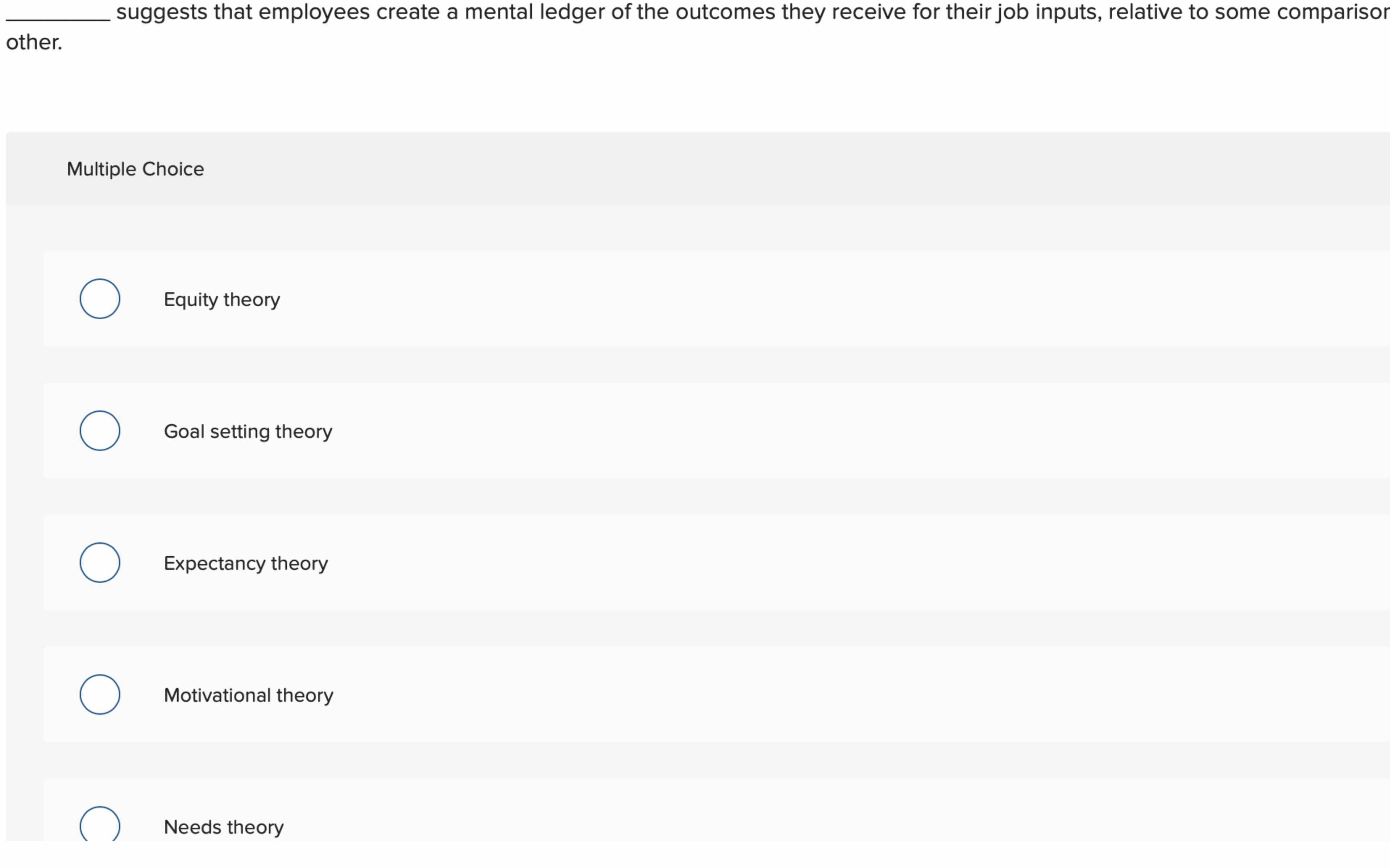This is a detailed screenshot of a computer monitor displaying a multiple-choice question about organizational behavior theories. The question reads: "___ suggests that employees create a mental ledger of the outcomes they receive for their job inputs relative to some comparison [cut off]." The possible answers, each preceded by a bubble for selection, include the following options:

1. Equity Theory
2. Goal-Setting Theory
3. Expectancy Theory
4. Motivational Theory
5. Needs Theory [cut off]

The question is partially obscured, particularly at the end, indicating that the full text might be cut off on the screen. The items listed are well-known theories related to employee motivation and behavior within an organizational setting.